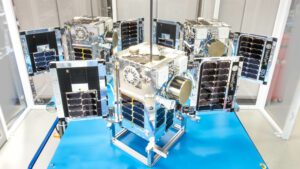The image depicts a laboratory setting with a variety of machinery on an aqua blue tiled floor, interspersed with a dark blue stripe and a blue carpeted area. At the forefront, there is a tall, box-like robotic device with a clear top that reveals its inner mechanics. This machine has a black and silver base equipped with drawer-like features, potentially for accessing internal electronics. Prominently, there's a large gold cylindrical or oval component, possibly a vent cover or knob, on the right side of the device. Surrounding this machine are other black and white machines, some with blue and light blue elements. The laboratory features white-outlined windows on the sides, with something red and wheeled faintly visible outside the right window. Tall black structures are visible in the background, adding to the complexity of the scene. There are no visible people, animals, or writings within the image.